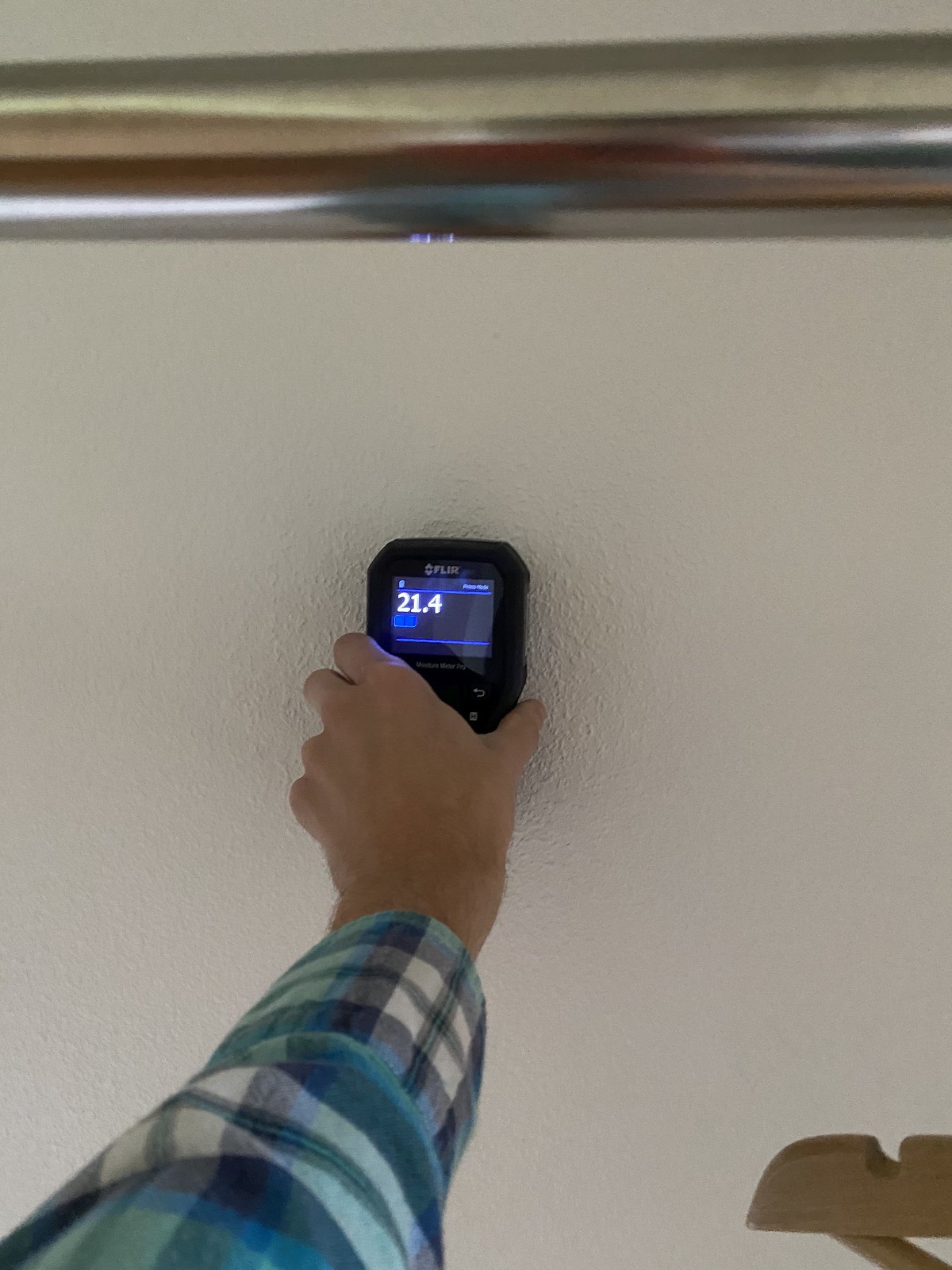In the photograph, a device bearing the label "FLIR" is pressed against a surface, which, based on the presence of a popcorn texture, is likely a wall or possibly a ceiling. The context suggests it is more likely a wall, as evidenced by a hanger visible in the lower right corner, appearing to be suspended in an upright position—fitting with the hypothesis that the machine is against the wall to comply with the principles of physics. The device displays a reading of 21.4, although its exact function isn't clear; it could potentially be measuring moisture. Further, a metal pole spans horizontally across the upper portion of the image, possibly supporting the hanger. The setting resembles a closet, considering the arrangement of these elements.